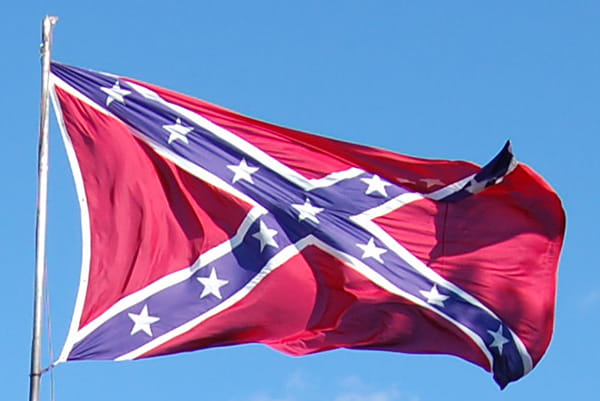The image showcases a Confederate flag flying high on a metal pole against a clear, cloudless blue sky. The flag, rippling in a stiff wind, features a vivid red background adorned with a prominent blue diagonal X, outlined with thick white lines. Each arm of the X is studded with white stars, which likely total around 14, extending towards each corner and converging at the center. Shadows cast by the waving fabric add depth and movement to the scene. The flag's entire design of intersecting blue bands and stars is crisply detailed, although parts of it are creased and bent due to the wind. This photograph captures the controversial symbol in stark clarity, evoking its historical and modern connotations.